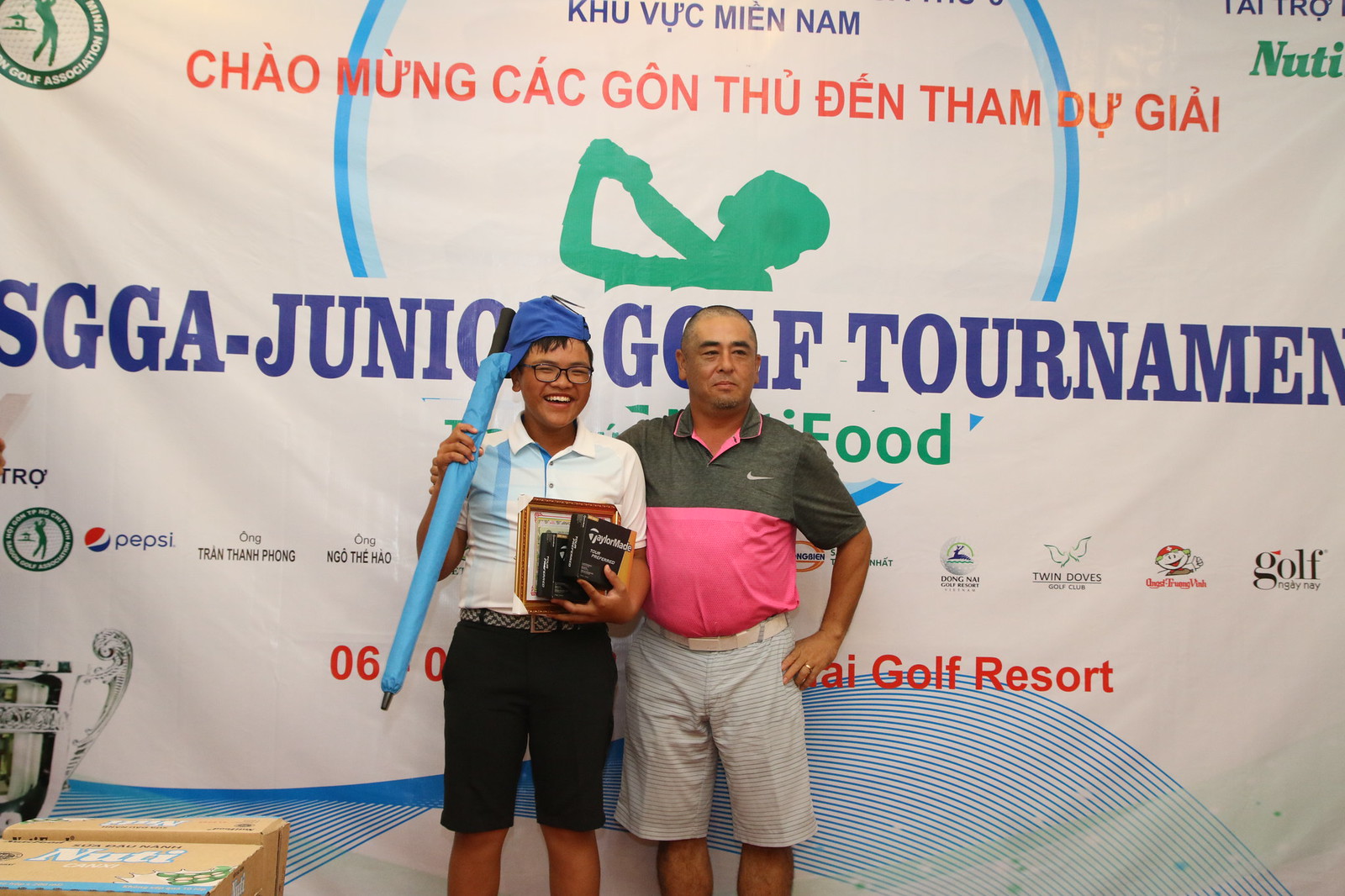In the photo, a young Asian male and an older man, possibly his father, stand proudly in front of a banner for the SGGA Junior Golf Tournament. The youthful boy, likely in his early teens, is beaming with excitement. He wears a blue hat, glasses, a white polo shirt tucked into black khaki shorts, and a checkered belt. In his hands, he holds a closed umbrella, two boxes, and a wood-framed picture. To his right, the older man, perhaps his dad, rests a hand on his shoulder. The father is dressed in a stylish gray and pink Nike polo shirt paired with striped white shorts and a white belt. The background features a white banner adorned with various logos, including Pepsi, indicating local sponsorships. A trophy is also visible to the side, reinforcing the celebratory atmosphere of the golf tournament event.